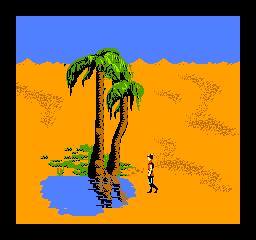In this animated, retro-style video game screenshot, the scene is set on a predominantly orange ground, speckled intermittently with brown patches, giving the terrain a textured appearance. A small, human-shaped character is depicted in a side view, standing near the center. In the foreground, a blue puddle disrupts the orange expanse, adding contrast to the scene. Flanking the puddle are two brown palm trees with lush green tops, rooted firmly in the digital soil and contributing to the vibrant environment. The background sky is a clear, light blue, enhancing the sense of openness in the setting. Encapsulating the entire image is a thin, black rectangular frame, which serves to focus the viewer's attention on the detailed landscape within.